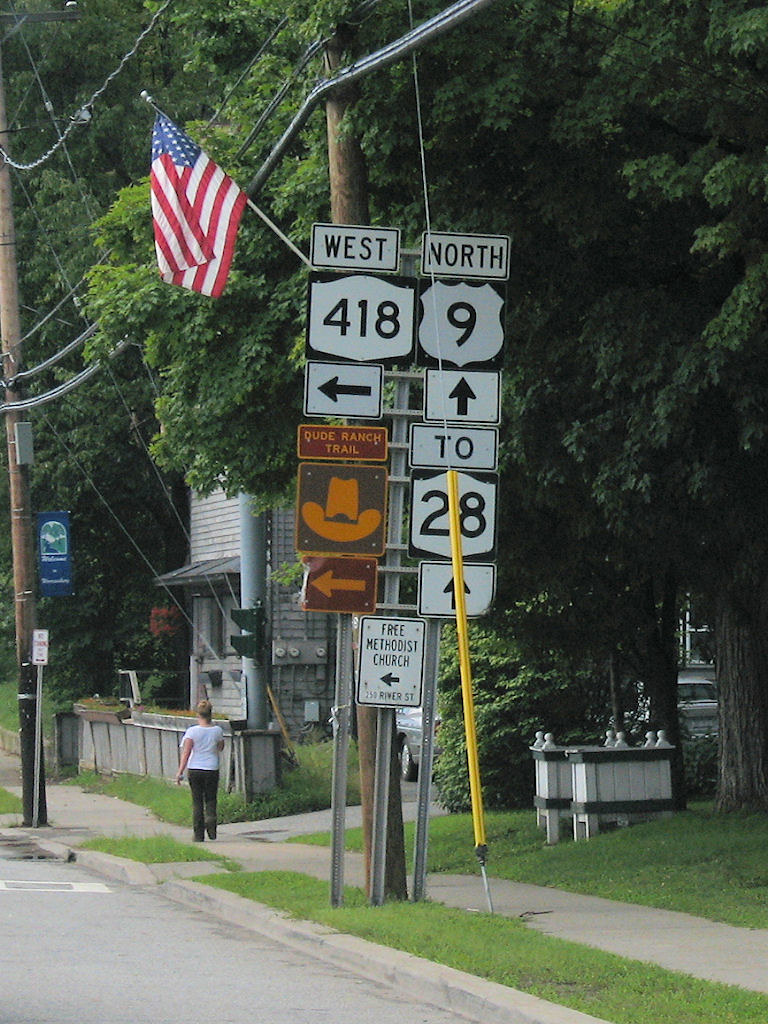In this vibrant, vertically-shot color photograph taken from the street, we look at a heavily-signposted metal pole situated on a grassy median to the right of the sidewalk. The pole is adorned with an array of traffic and navigational signs, each offering varied guidance. At the top, a sign directs travelers towards "North 9" and "28" straight ahead, while another directs towards "West 418" with an accompanying rectangular sign pointing left. There's also a prominent rectangular white sign indicating "FME Methodist Church" with a black arrow. Beneath this, a brown rectangular sign with orange lettering highlights the "Dude Ranch Trail" accompanied by a distinctive yellow cowboy hat emblem and another left-pointing arrow.

Adjacent to this signpost, a woman in a white shirt and dark pants strolls along the gray, well-maintained sidewalk flanked by thick concrete curbs and lush green park strips. Further into the background, there are several houses with an old-fashioned charm, reminiscent of a quiet, idyllic town. A bus stop and an American flag, which appears to be mounted on a pole attached to the power line, can also be seen. Tall trees with ample foliage add a sense of tranquility to the scene, contrasting the utility and direction provided by the myriad of signs.